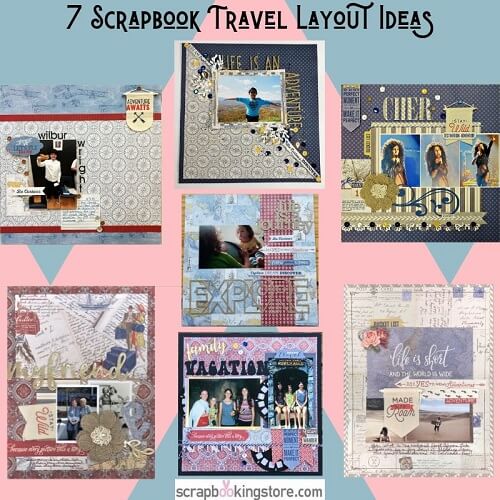The image is a detailed, square-shaped book cover titled "Seven Scrapbook Travel Layout Ideas" in bold black letters at the top, set against a predominantly light blue background with pink accents. This creative cover showcases seven distinct scrapbook layout ideas arranged in a visually appealing manner. Each layout is intricately designed with a mix of photos and decorative elements.

In the upper right panel, there is an image featuring Cher, with the word "Cher" prominently displayed alongside the phrase "In the perfect moment, make it perfect." To the left of this, a woman stands with arms outspread under the caption "Life is an adventure." Below this, a photo depicts a person holding a baby, and it carries the inspirational message "Life is a journey, explore."

The bottom middle panel highlights a family vacation, showing a series of photos of the same three girls at different ages and stages of life, complemented by the word "Vacation" in big, bold letters. In the lower left corner, an elderly couple is seated, and above them, there’s an inscription that reads "My Friend" with a checkmark. Lastly, in the lower right panel, the image contains the phrase "Life is short, and the world is wide."

All the scrapbook covers are arranged in a grid with two columns on the left, three in the middle, and two on the right, creating a balanced and engaging overall layout.